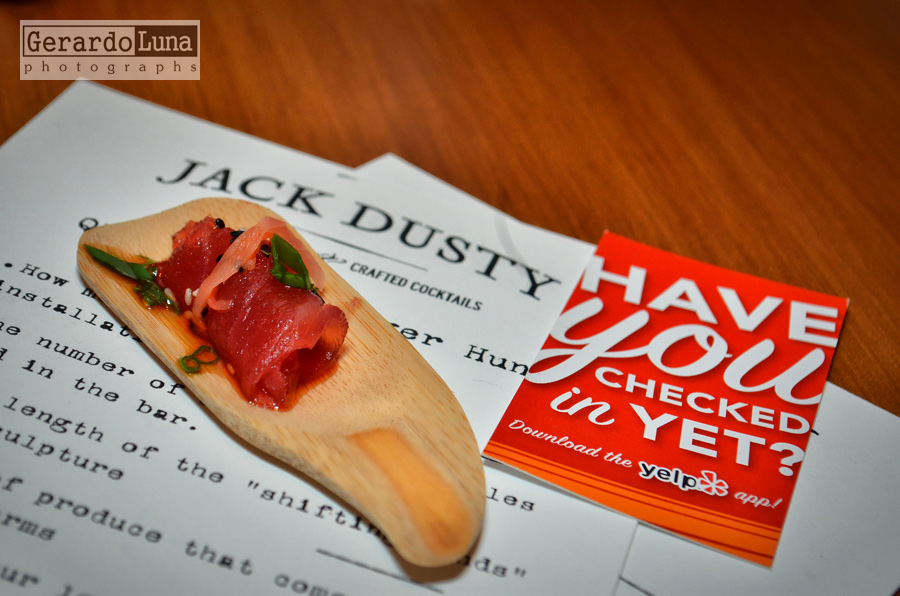In this photograph, we see a carefully arranged setting featuring a piece of tuna sashimi, elegantly displayed on a small wooden serving piece that resembles a mini tray or spoon. The tuna is wrapped into a cylindrical shape, garnished with chives, and possibly a hint of sauce, adding a touch of greenery. This setup rests atop some white papers marked with "Jack Dusty" in a stylish font, followed by "Crafted Cocktails," which hints at the possible setting being a bar or a restaurant known for its cocktails. A smaller red piece of paper next to the wooden surface carries an advertisement prompting viewers to "Have you checked in yet? Download the Yelp app." The scene is set on a dark wooden table, adding contrast, and in the upper left corner, there is a logo reading "Gerardo Luna Photography," with 'Gerardo' on a white background and 'Luna' on a black background, giving credit to the photographer of this meticulously crafted culinary presentation.